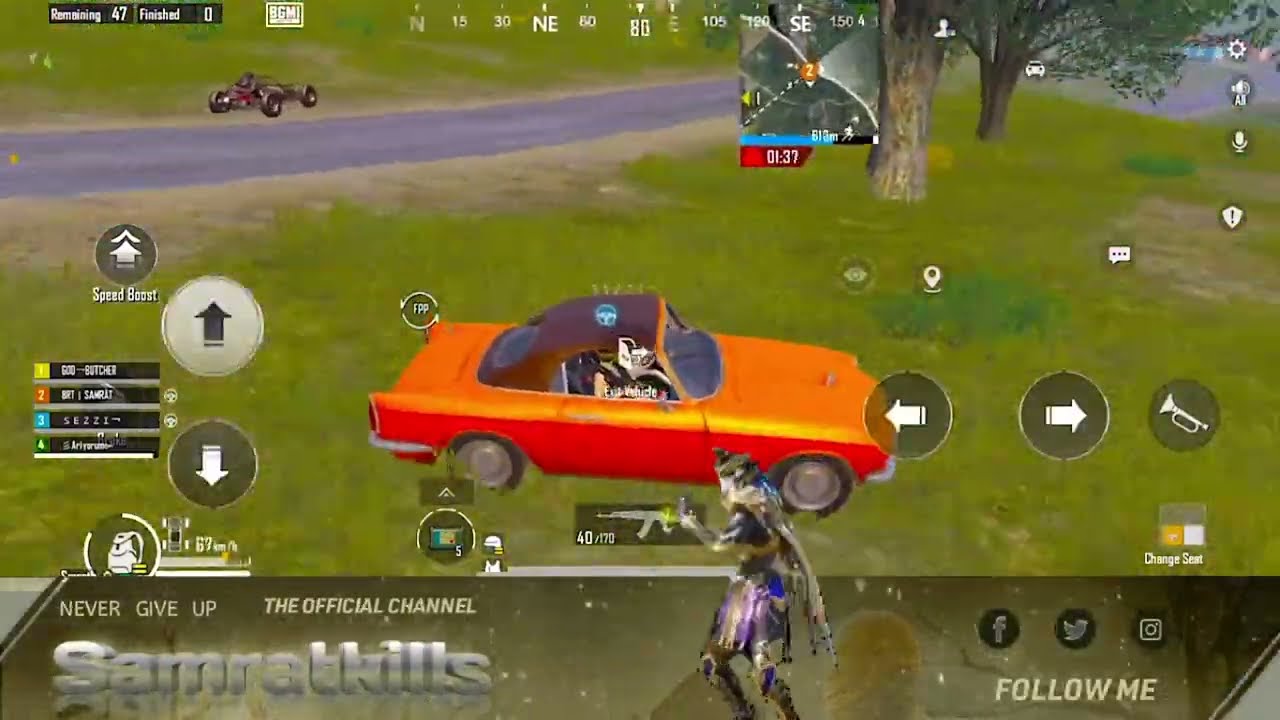The image is a screen capture from a video game, displaying a vibrant park-like setting with a rich green background. Dominating the center is an orange sports car reminiscent of classic MG models, featuring a black ragtop convertible and black wheels with gray hubcaps. Surrounding the car are various directional arrows—up, down, left, and right—which suggest movement options within the game. Particularly notable is an arrow labeled "super boost" and an icon featuring a trumpet. In the distance, a small race car can be seen on a long gray track that cuts through the scene from left to right, adding a sense of depth.

The scene also includes two tree trunks situated above and to the right of the car, further enhancing the park-like atmosphere. At the top of the screen, there is a compass with a mini-map, providing additional navigation information.

The bottom section of the screen is covered by a gray banner with white text that reads, "Never Give Up, The Official Challenge, Samrak Kills." To the right of this message are social media icons for Facebook, Twitter, and Instagram, accompanied by the text "Follow Me." Adding to the game's immersive interface, a character in gray is visible below the car, facing left and seemingly holding a gray or silver firearm. The rectangular image, wider than it is tall, encapsulates a dynamic and interactive gaming experience packed with details and various in-game elements.